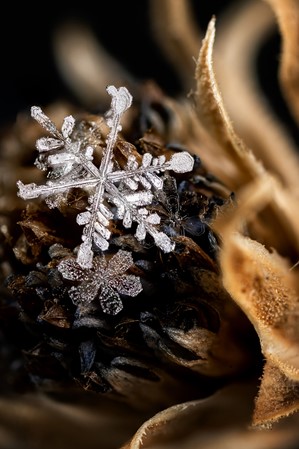This is a color photograph featuring an extreme close-up of a delicate, star-shaped snowflake with intricate, leaf-like patterns and hexagonal lines at its center. The snowflake, shiny and icy, spans about three inches along each of its six arms. It is positioned above a smaller, floral-shaped snowflake, both of which rest on a dark, ambiguous object partially resembling a black or brown pine cone or seed. To the right, a light brown stem or seed pod is visible. The background of the image is blurry, predominantly black and brown, providing a stark contrast to the meticulously detailed and seemingly digitally crafted snowflakes. The composition of the photo is much taller than it is wide, focusing solely on these natural elements without any presence of people, animals, or man-made structures.